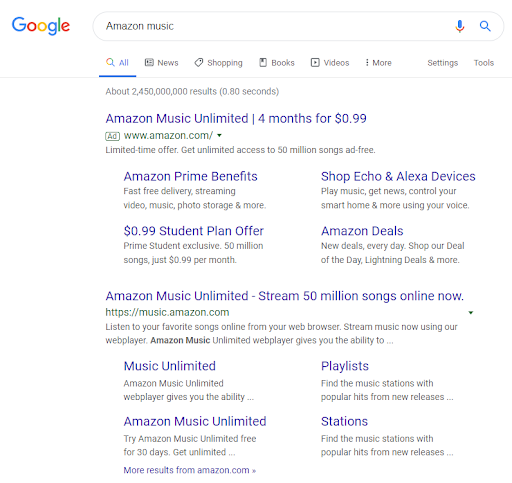Here's a detailed and cleaned-up descriptive caption for the image:

---

The image depicts a search being conducted on Google's homepage, which features a pristine white background. In the upper left corner, the iconic Google logo is displayed in its traditional colors: blue, red, yellow, blue, green, and red. Below the logo, about an inch from the left edge, there's a search bar that spans across to the right side of the page.

Inside the search bar on the left side, the text "Amazon Music" is typed in black. To the right, there is a blue search icon followed by a blue voice search icon. 

Directly beneath the search bar, on the left side, the word "All" is displayed in blue with a blue underline, indicating the selected search category. Adjacent to it are the category labels "News" (with a news icon), "Shopping" (with a shopping icon), "Books" (with a book icon), "Videos" (with a video icon), and "More" (with an additional options icon), all in black font. To the far right, there are the "Tools" option and the "Settings" option, again in black.

Further down, the search results are presented. The text indicates the number of search results and the time taken to retrieve them. The first result displays "Amazon Music Unlimited" in purple, followed by an offer of "Four months for $0.99," separated by a dividing line. Below this, "Ad" is written in green, accompanied by the Amazon link "www.amazon.com" in green as well. There is a brief description in black beneath this link.

Subsequent sections feature additional information: "Amazon Prime Benefits" in purple with two lines of description in black, "Shop Echo and Alexa devices" with two lines of text under it, "99¢ student plan offer," and "Amazon deals," each followed by respective details.

Further results include a link labeled “Amazon Music Unlimited - Stream 50 million songs online now.” Below this, "Amazon.com" appears in green, accompanied by two descriptive lines. On the left side, titles such as "Music Unlimited" and "Amazon Music Unlimited" are bolded, while the right side mentions specific features like "Playlists" and "Stations," with additional details presented in two lines of text underneath.

---

This description provides a comprehensive overview of the visual layout and contents of the search results on Google's homepage for "Amazon Music."